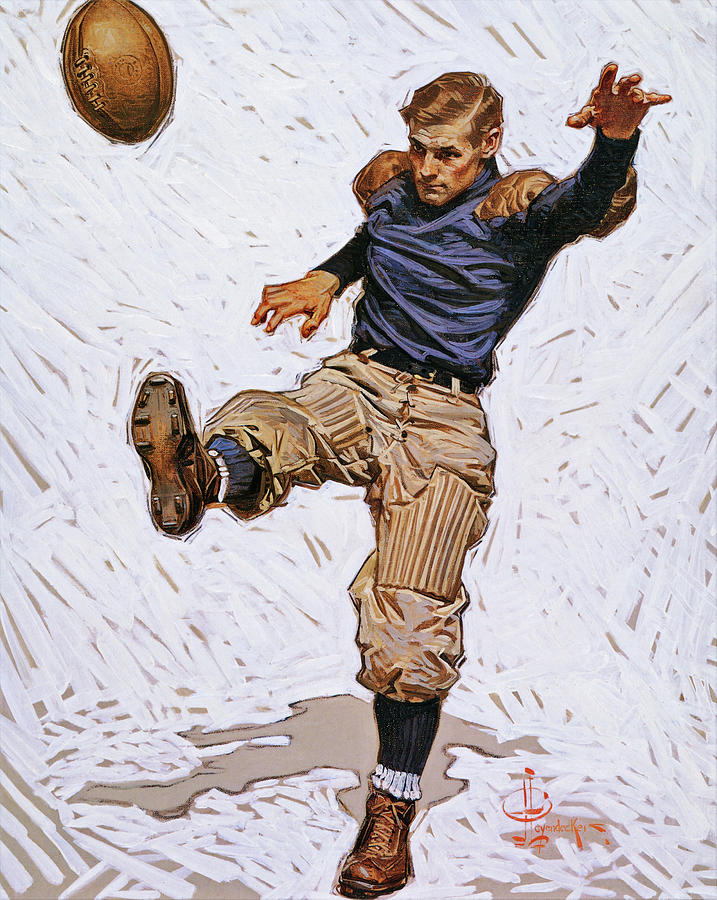This detailed illustration by J.C. Leyendecker portrays an old-fashioned football player, potentially from the 1920s, during a punt. The athlete, a white man with short brown hair combed to the side, strikes a focused pose with furrowed brows while facing the viewer at a slight angle. He sports a blue long-sleeve shirt featuring brownish shoulder and elbow pads, light brown pants, and dark knee-high socks paired with brown shoes. His left arm is outstretched in front of him, and his right arm is slightly bent with the hand down near his waist. The right leg is raised, having just kicked a football or perhaps a rugby ball, which is visible in the upper left-hand corner of the image. Notably, he lacks a helmet, emphasizing the nostalgic feel of the artwork. The background showcases abstract strokes of white paint, adding a dynamic, artistic flair to the scene. A possible logo or inscription, "Cynodex," can be faintly discerned in the lower right-hand corner. Overall, this piece captures a vintage sporting moment with a striking mix of detail and abstraction.